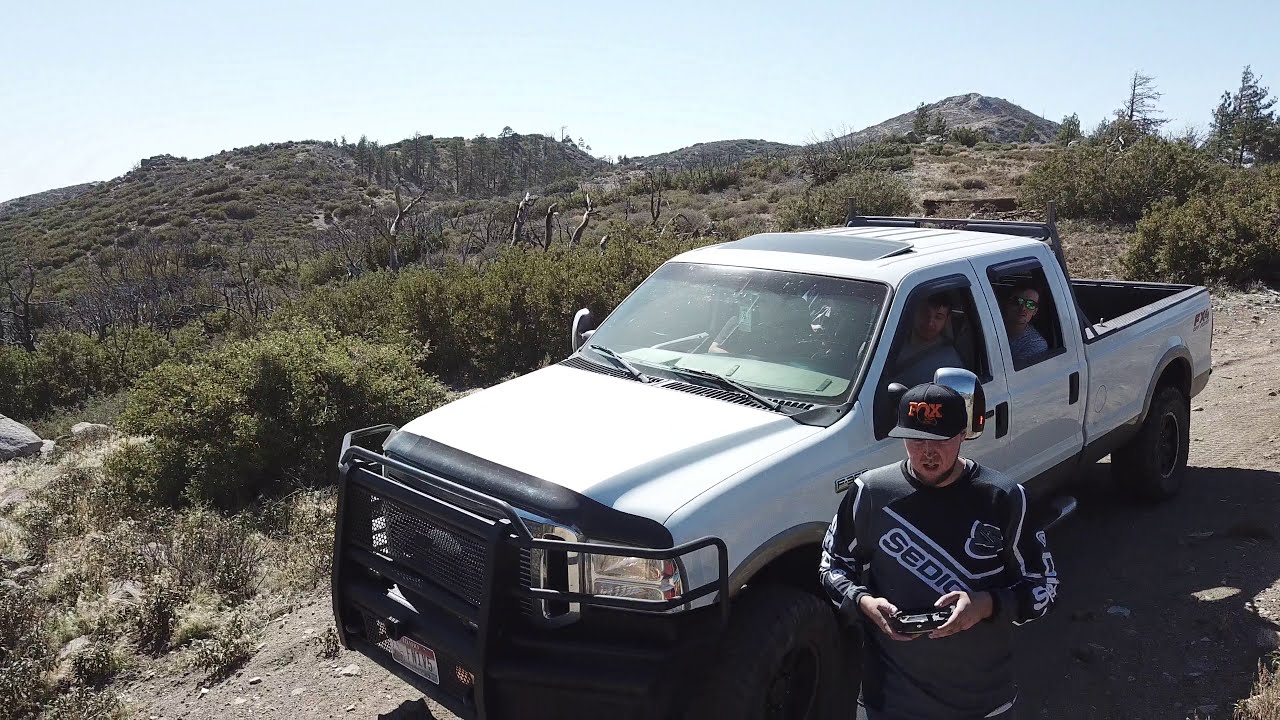The image captures a white Ford pickup truck equipped with a large police bumper and black wheels, parked on a dirt road in a desert-like setting. The truck has a sunroof and four doors, with two men visible through the open driver's side windows—one in the front seat and another in the back, the latter wearing sunglasses. Standing to the left of the truck is a man dressed in a black and gray long-sleeved shirt, a black cap with orange print, and a black jacket that has "S-E-D-I-C" written in white letters on the front. He is focusing intently on a device, which might be a cell phone or GPS, in his hands. The surrounding landscape is characterized by green brush, cacti, bare small trees, and dirt-covered hills, with one prominent hill resembling a small mountain in the background. The bright, sunny sky illuminates the entire scene.